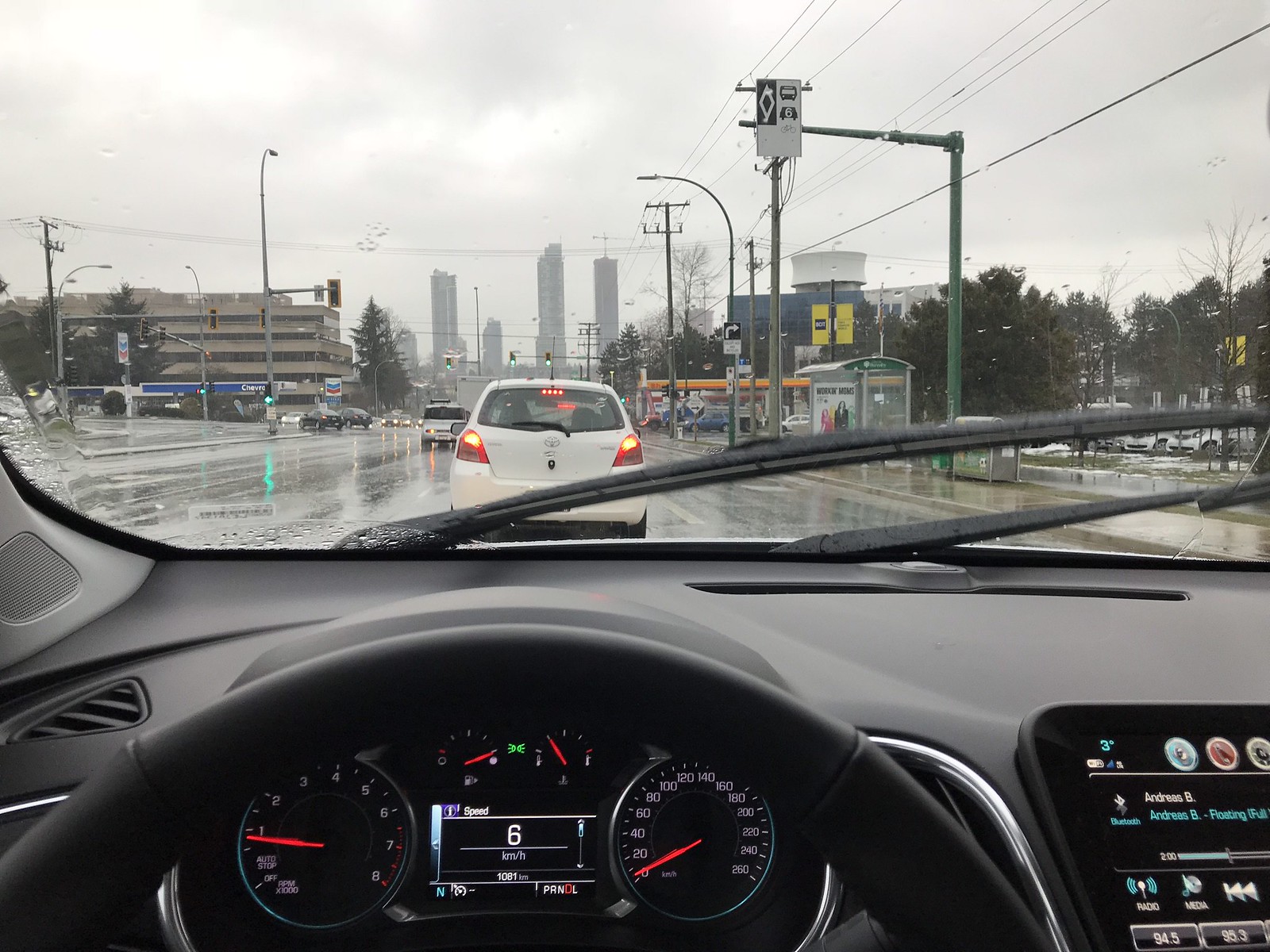A detailed photograph taken from the interior of a modern vehicle on a rainy day. The dashboard, illuminated and displaying a low RPM and a speed of six kilometers per hour, indicates the car is fairly new with an odometer reading of 1001 kilometers. The automatic transmission is in drive, as evidenced by the red indicator on the "D" of the PRNDL display. Additional gauges show the fuel tank nearly full and the oil pressure at the first notch out of five. A traditional round speedometer with a red needle also confirms the vehicle's speed. 

The photograph is centered on the steering wheel and dashboard, with a display to the right showing text, possibly the music the driver is listening to. Through the rain-speckled windshield, a city scene is visible with tall buildings, trees, a bus stop, and a white car ahead with its brake lights illuminated.